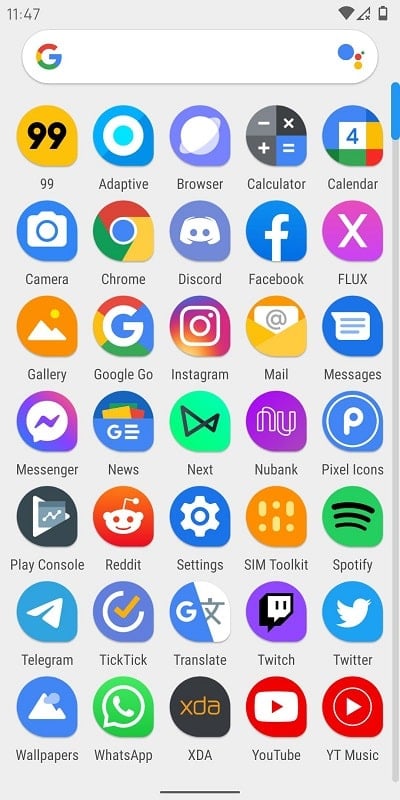The screen capture features the home screen of a cell phone, displayed against a gray backdrop. At the top left corner, the time is shown in light gray as 11:47. On the top right, the Wi-Fi icon indicates a weak connection with only one bar, and the battery icon shows approximately 25% remaining charge.

Beneath the status bar is the Google Assistant search widget, identifiable by a multicolored Google 'G' on the left and the Google Assistant bubbles on the right. 

The main portion of the screen contains a grid of application icons arranged in seven rows and five columns. The icons, stylized like guitar picks with the pointy area positioned at the four o'clock mark, include the following apps from left to right, row by row: 99, Adaptive, Browser, Calculator, Calendar, Camera, Chrome, Discord, Facebook, Flux, Gallery, Google Go, Instagram, Mail, Messages, Messenger, News, Next, New Bank, Pixel Icons, Play Console, Reddit, Settings, Sim Toolkit, Spotify, Telegram, TickTick, Translate, Twitch, Twitter, Wallpapers, WhatsApp, XDA, YouTube, and YouTube Music.

At the very bottom of the screen, a darker gray line adds a subtle contrast to the background.